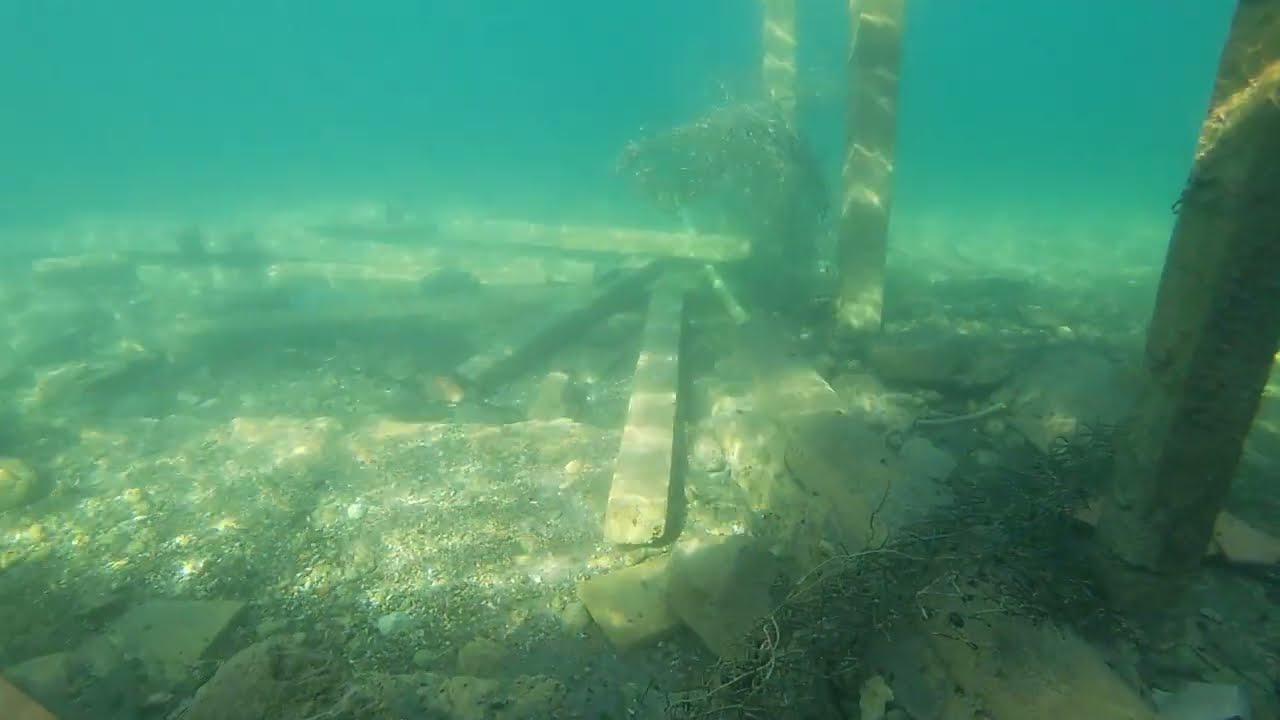The image depicts an underwater scene at what appears to be the shallow bottom of a large body of water, possibly an ocean. The water is tinted with shades of green and blue, suggesting a presence of algae or plankton. Scattered throughout the scene are pieces of wood and possibly metal debris, giving the floor a sparse and cluttered look. On the right side of the image, three upright poles are visible, likely the support beams of a pier or dock overhead. There is noticeable sunlight reflecting on the flat seabed, indicating the water is not very deep. The area lacks visible marine life such as fish, coral, or other plants, aside from some plant-like matter that is dark and not vividly green, adding to the murky and desolate atmosphere.